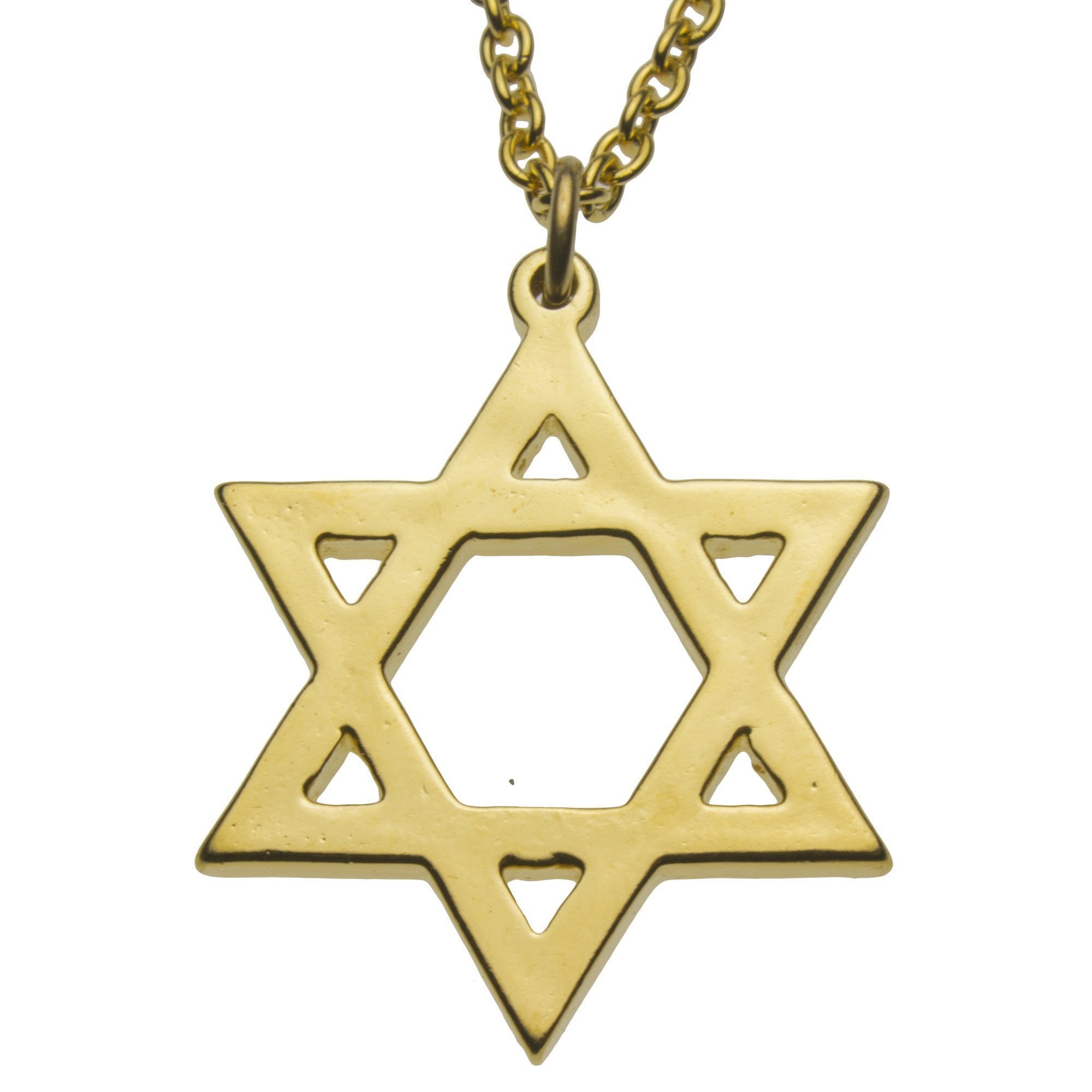The image showcases a close-up of a gold link necklace with a Star of David pendant. The pendant, a six-pointed star formed by overlapping two isosceles triangles, exhibits a detailed open design with a hexagon in the center and triangular cutouts at each point. The pendant, seemingly crafted from a metal plated with a gold alloy, contrasts with the duller gold of the chain, which appears to be brass. The composition is centered, with the necklace chain cut off right as it starts, set against a white background. The pendant casts a subtle shadow, suggesting it is a rendered image since the chain lacks a corresponding shadow. The overall image appears zoomed in, magnifying the pendant which is actually about the size of a marble. Despite its subdued shine, the intricate Star of David charm adds a touch of flashiness to the piece.